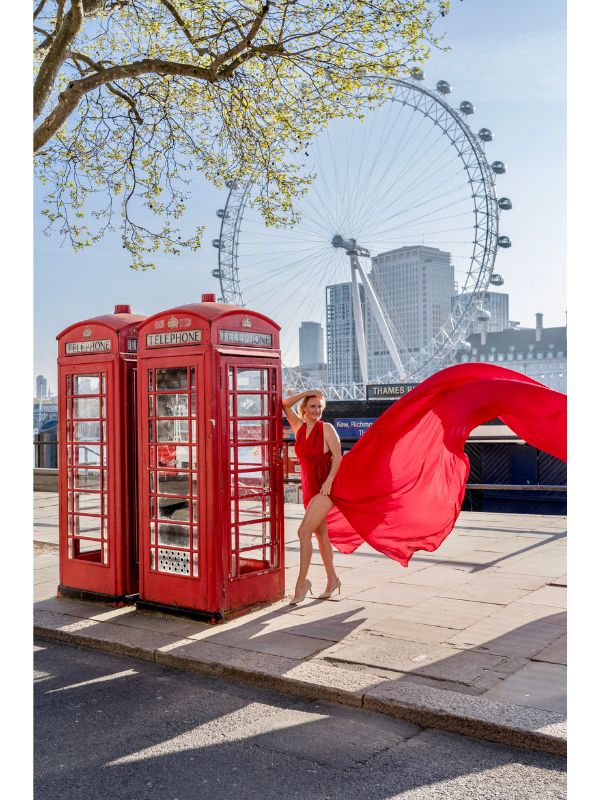In the image, a light-skinned woman in a flowing, sleeveless red dress is posing elegantly on a wide city sidewalk. The dress, dramatically caught by the wind, billows to the right, adding a dynamic element to the scene. She leans casually on one of two iconic red London telephone booths, using her right elbow for support while her hand sweeps through her hair. Set in portrait mode, the photograph captures the bustling ambiance of London during the day. To the left, a massive tree with yellow leaves branches out across the image, offering a natural contrast to the urban elements. Behind her, a sign reading "THAMES" hints at the river nearby, and in the background, the famous London Ferris Wheel stands tall, framed by several skyscrapers. The top right corner of the image reveals a clear blue sky, adding to the vibrant atmosphere of the scene.